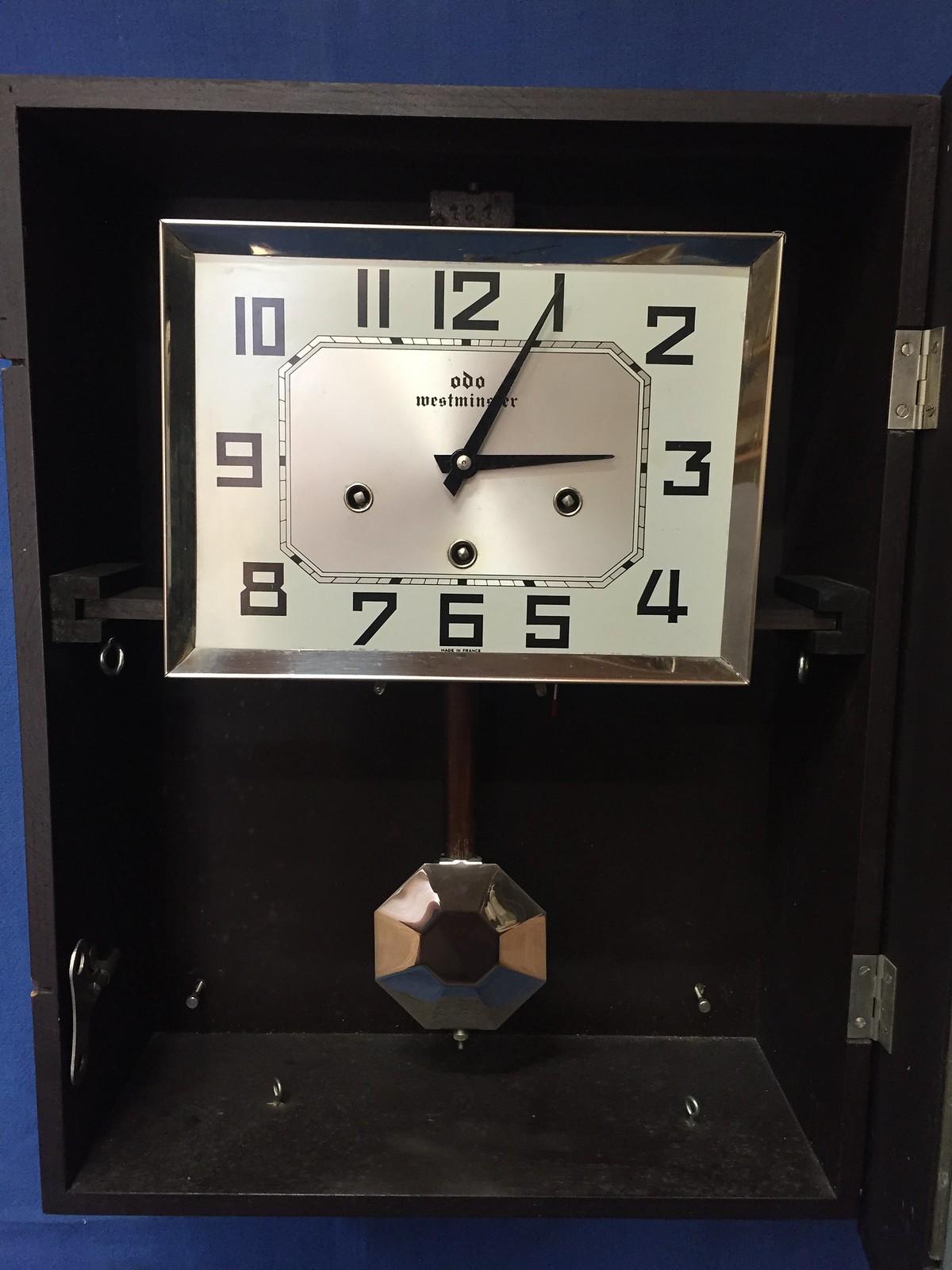A vintage wall clock from the 1950s or 1960s is showcased within an open cabinet box. The hinged right side of the box is visible, though the door itself is out of frame. The clock face, set within a rectangular chrome frame, features Arabic numerals and classic clock hands. The brand names "Odo" and "Westminster" are prominently displayed on the dial. Below them, an octagon-shaped pendulum hangs, adding to the clock's distinctive retro charm.